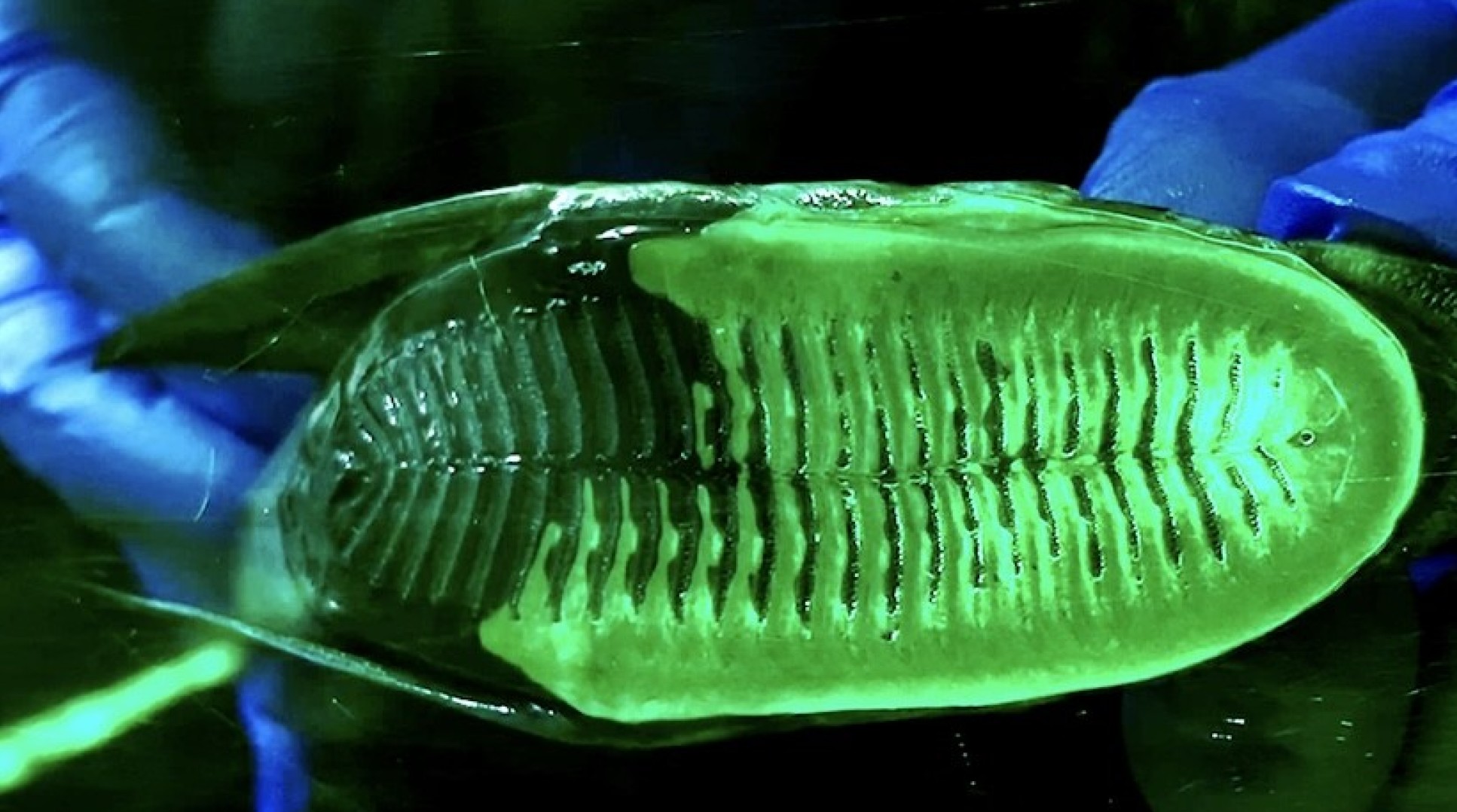The photograph features a close-up view of the bottom of a shoe sole, predominantly vibrant neon green with some darker forest green accents. The sole appears to be made of a gel material and exhibits dark creases that resemble tread patterns. Flanking both sides of the sole are two royal blue tubes, which are reminiscent of long balloons or rolled-up cloths. The background is a very dark black, punctuated by small white flecks near the top and bottom, and slightly blurred bright blue objects towards the left and upper right. In the upper section of the shoe sole, there are pointed green features that are suggestive of leaves or a plant-like structure. At the center, the sole's textured treads form a repetitive pattern that accentuates the design. Amidst the neon green, a smaller, lighter green section is visible at the bottom left, which looks akin to a stem. The combination of these vivid colors against the dark background creates a striking and memorable impression.